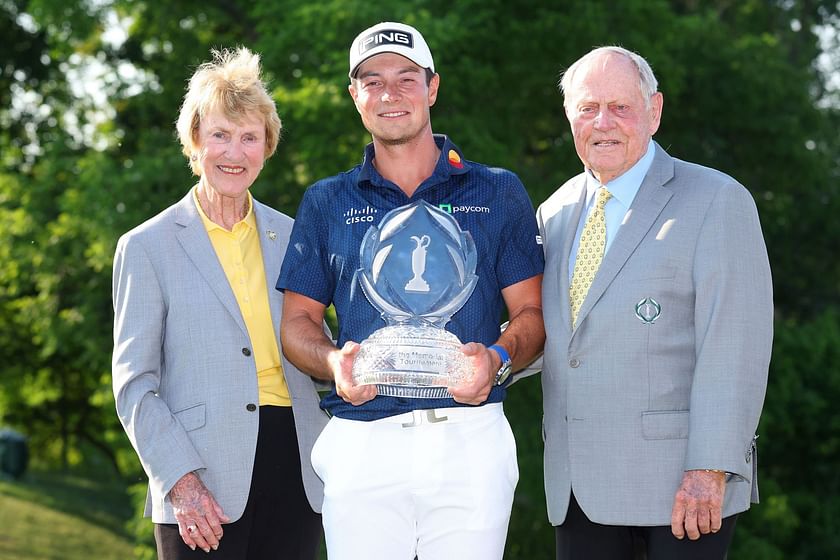In this outdoor photograph, a younger man stands at the center, proudly holding a glass golf trophy with an inscription on its base that includes the word "tournament." He wears white pants and a blue button-up shirt featuring the logos of Cisco and Paycom, complemented by a white Ping cap. Flanking him on either side are two older individuals. To his left is a woman with short blonde hair, dressed in a gray open blazer over a yellow button-up shirt and black pants. On his right stands an older man with gray hair, attired in a gray business suit, a white undershirt, a yellow necktie, and black pants. Both older individuals have their arms affectionately around the young man. The backdrop of the image features lush green grass and trees, emphasizing the outdoor setting, likely a golf course.